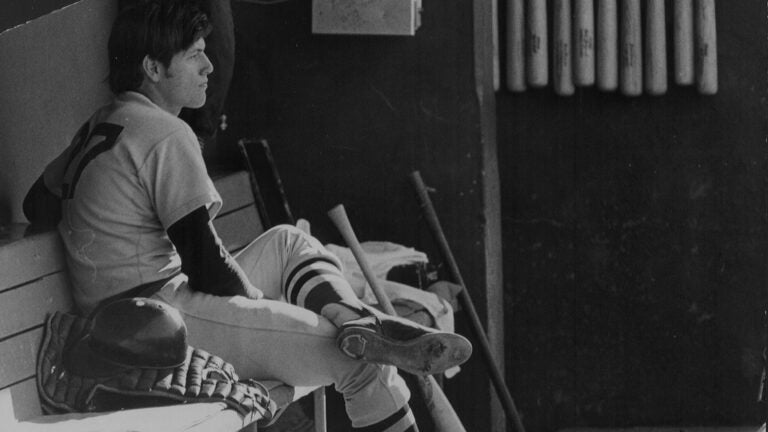In this evocative black and white photograph, a lone baseball player, identified by the number 27 partially visible on his back, sits pensively on a wooden bench in a dugout. The scene is imbued with a sense of solitude and contemplation. The player sits with his left ankle resting on his right knee, gazing out to his right as if observing the ongoing game with a mixture of concern and disappointment. He dons a traditional baseball uniform—white with black sleeves—and his black hair and the detailed stitching of his outfit are clear despite the image's slightly soft focus. Next to him on the bench lies a black helmet and what appears to be a catcher's mitt, indicating his role on the team. Two baseball bats rest nearby, and the backdrop reveals a row of wooden bats hanging from the top edge of the dugout, which fades into deep shadows. The overall atmosphere is one of introspection, capturing the player's solitary moment amidst the unseen commotion of the game.